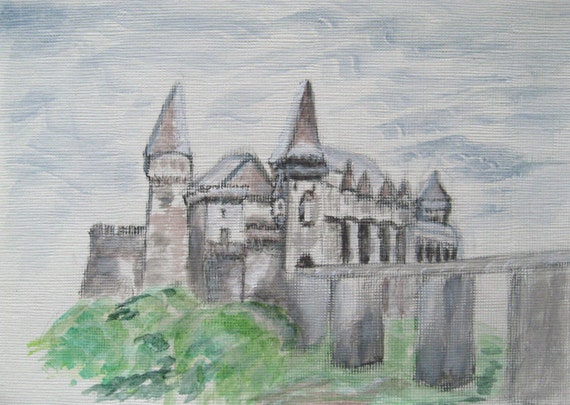This image is a rectangular canvas painting, about four inches wide and three inches high, depicting a medieval stone castle with a mixture of gray and brown hues. The castle, which exudes an elegant yet somber feel, features multiple towering structures, including pointed towers and watchtowers. Vertical columns and pillars are prominently supporting the front facade of the castle. A bridge, composed of similar brownish-gray tones with hints of white, extends across a green moat or grassy bank towards the lower right-hand corner of the canvas. Below this bridge, additional green vegetation is visible. The hill beneath the castle slopes downward towards the left, blending into the greens and blues, enhancing the landscape. Above the castle, the sky is rendered in grayish-blue squiggles, suggesting clouds amidst a blue backdrop. The overall faded style of the painting, with visible canvas lines suggesting watercolor technique, adds a touch of vagueness, enhancing the medieval and somber aesthetic.